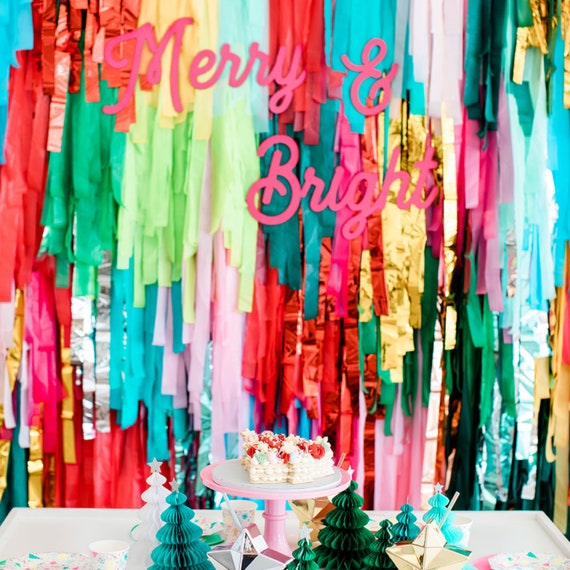This somewhat blurry, nostalgic Christmas photograph captures a festive scene filled with vibrant decorations. The focal point is a white table set with a pink cake stand holding a cake decorated with colorful flowers. Surrounding the cake are mini pavlova desserts, paper plates, and cups, all set against a rainbow of streamers cascading down from above. These streamers, made of various materials—some shiny and plastic, others paper—create a lively backdrop with colors ranging from red, green, yellow, blue, to gold and white. Amidst the streamers, a hot pink cursive sign cheerily proclaims "Merry and Bright." Additionally, the table is adorned with paper ruffled Christmas trees in shades of green and white, enhancing the holiday spirit of the scene, making it a perfect setup for a Christmas party photo booth.